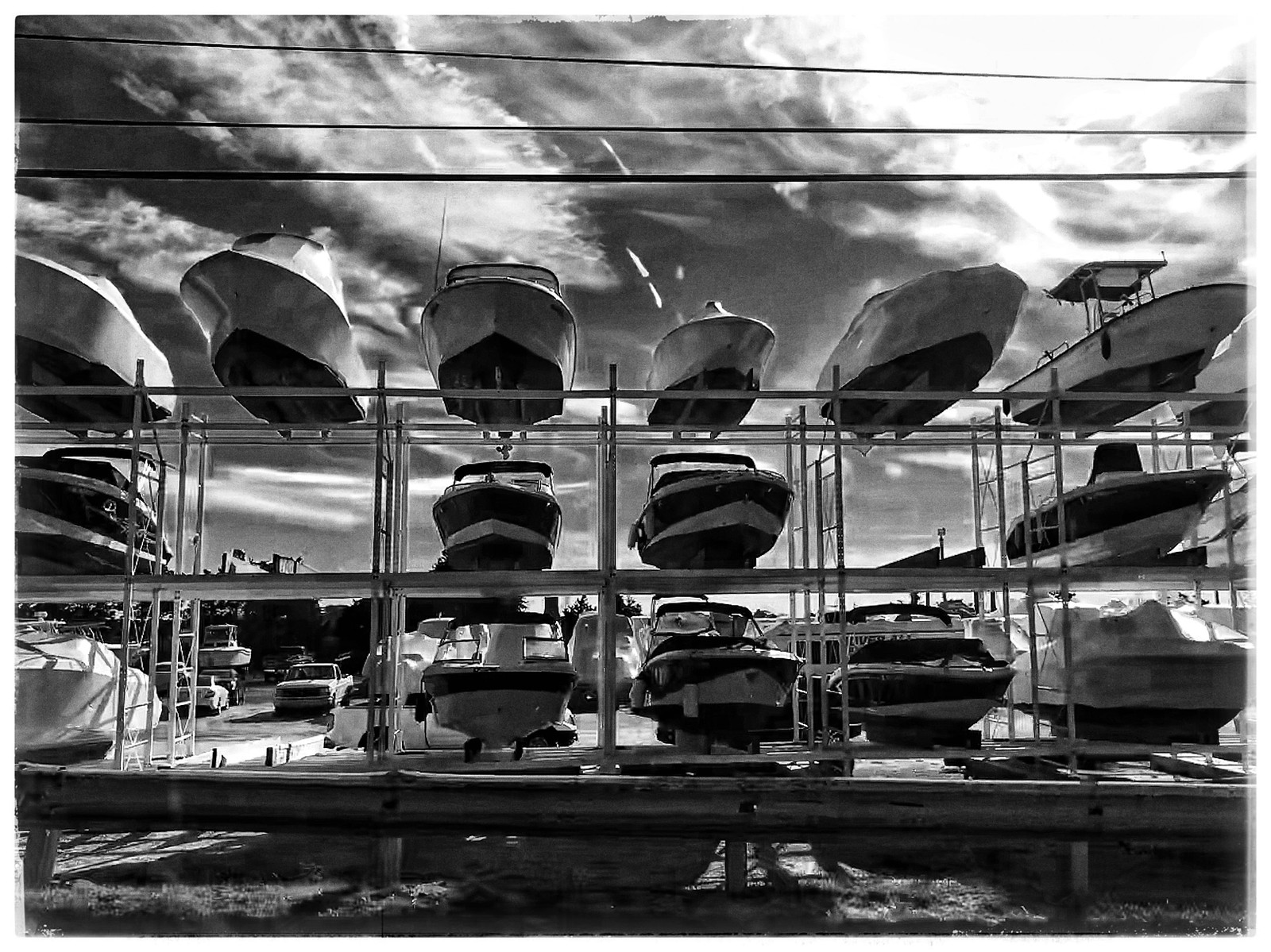This black and white photograph captures a detailed scene at a dry boat storage facility set against a dramatic, cloud-filled sky. In the foreground, a multi-tiered metal structure with large shelves holds a series of motorboats. These white, personal-sized boats, some with covers, are neatly arranged on the three levels: the top shelf has 6 boats, the middle shelf has 4 with 2 empty spots, and the bottom shelf holds 5 boats with one open slot. The structure sits on a wooden dock by the water, and in the background, there is a hint of a truck and more boats hitched to vehicles, suggesting additional boat activity. The intense contrast of the clouds highlights the sunny day, creating a striking interplay of light and shadow.